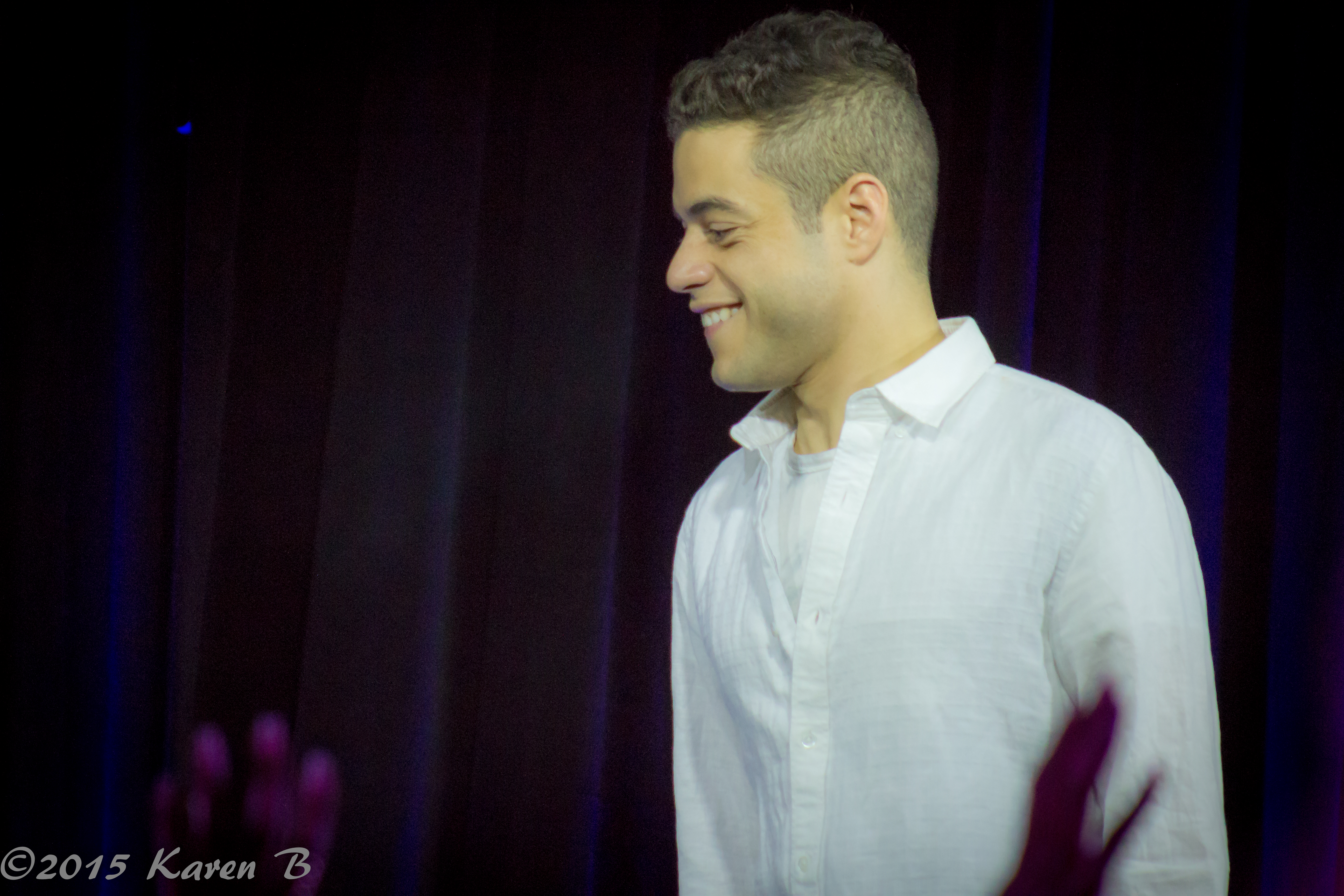The photograph is a color image in landscape orientation, capturing actor Rami Malek positioned slightly to the right of center in profile, facing left. He is smiling and clean-shaven, with an undercut hairstyle where his short brown hair is shaved close on the sides and back. He is dressed in a slightly see-through button-up white shirt with white buttons, worn over a white crew-neck short-sleeve t-shirt. The background features a rippling blue fabric curtain that spans the entire backdrop. In the bottom left of the image, a semi-transparent white text reads, "Copyright 2015, Karen B." The foreground reveals the fingertips of multiple off-screen individuals, as though they are waving or raising their hands. Additionally, the bottom left corner contains some out-of-focus elements that resemble small purple flowers, while a shadow of a person's hand is noticeable in front of Rami's shirt sleeve on the right side. The photograph is a representation of realism.